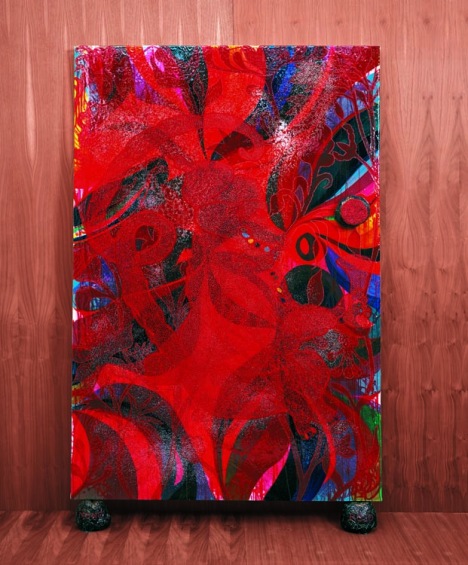The image features an abstract piece of artwork that dominates most of the frame. This artwork, resembling a painted canvas or possibly a decorated paper bag, is resting on what appear to be two dark objects—perhaps ornately painted blue-green balls, black rocks, or rollers—positioned underneath on either side. The background consists of a cherry-colored wooden wall and a floor made from thin wooden boards, some with visible cutouts.

The canvas itself is taller than it is wide and brims with vibrant, swirling patterns and colors. The primary colors include bold reds, dark blues, and blacks, with notable swirling and dripping effects. The central area consists of a striking red color, overlaid with darker red patterns. Surrounding this central red area are various shapes and swaths of blues, greens, and yellows, with these bright accents concentrated towards the edges—greens particularly towards the bottom right and yellows at the upper left and middle right sections. The overall effect is a visually stimulating, complex blend of abstract shapes and colors.